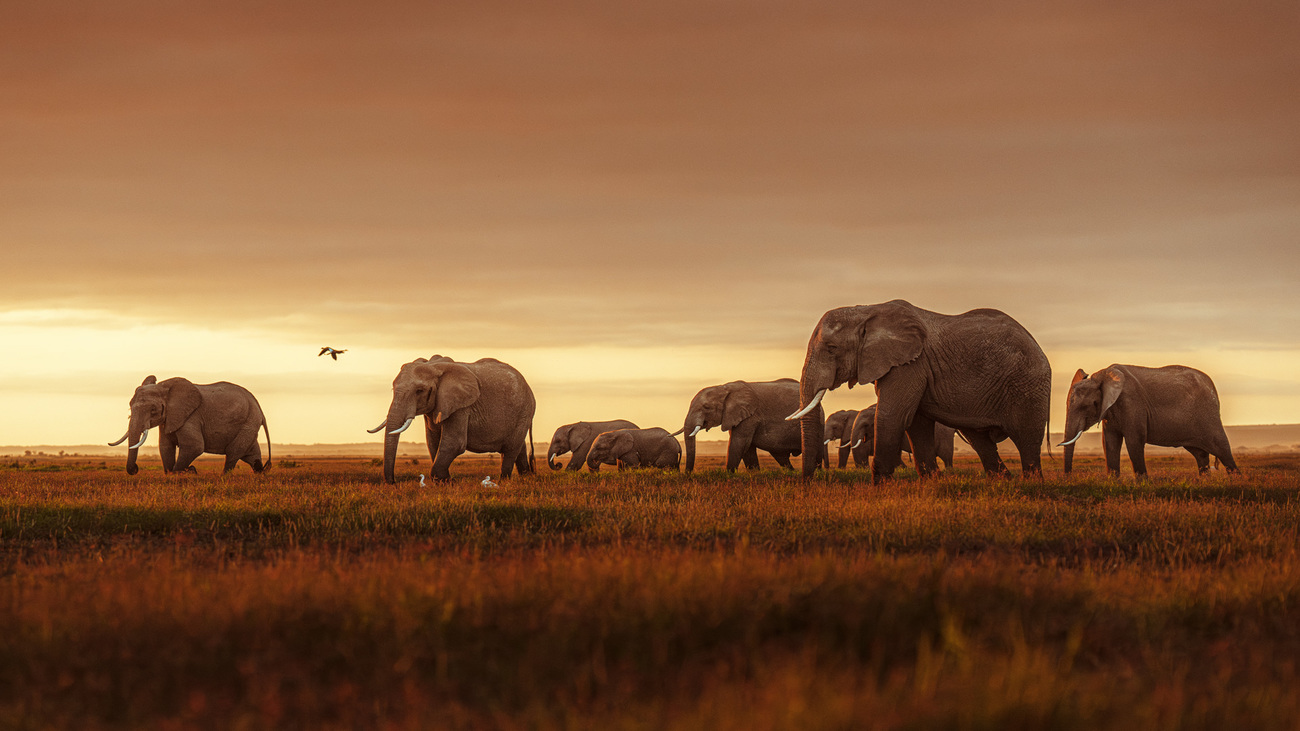The image captures a breathtaking scene on an African Plain at either sunrise or sunset, with a vibrant orange horizon that lights up the flat landscape, making the grasses glow in shades of orange. The sky above is dominated by dark clouds, suggesting an impending storm, which provides a dramatic contrast to the bright colors near the horizon. In the middle of this serene landscape, a herd of nine elephants is seen migrating slowly from right to left. The lead elephant, with its head down, is followed by eight others, some of which are noticeably younger and smaller. Their dark, brownish bodies contrast starkly against the sunlit grasses, and their white ivory tusks are prominently visible. To the top right, a single bird soars in the sky, while some white birds are also seen on the ground near the elephants. The tableau evokes the timeless rhythm of nature, accentuated by the warm glow of the setting or rising sun.